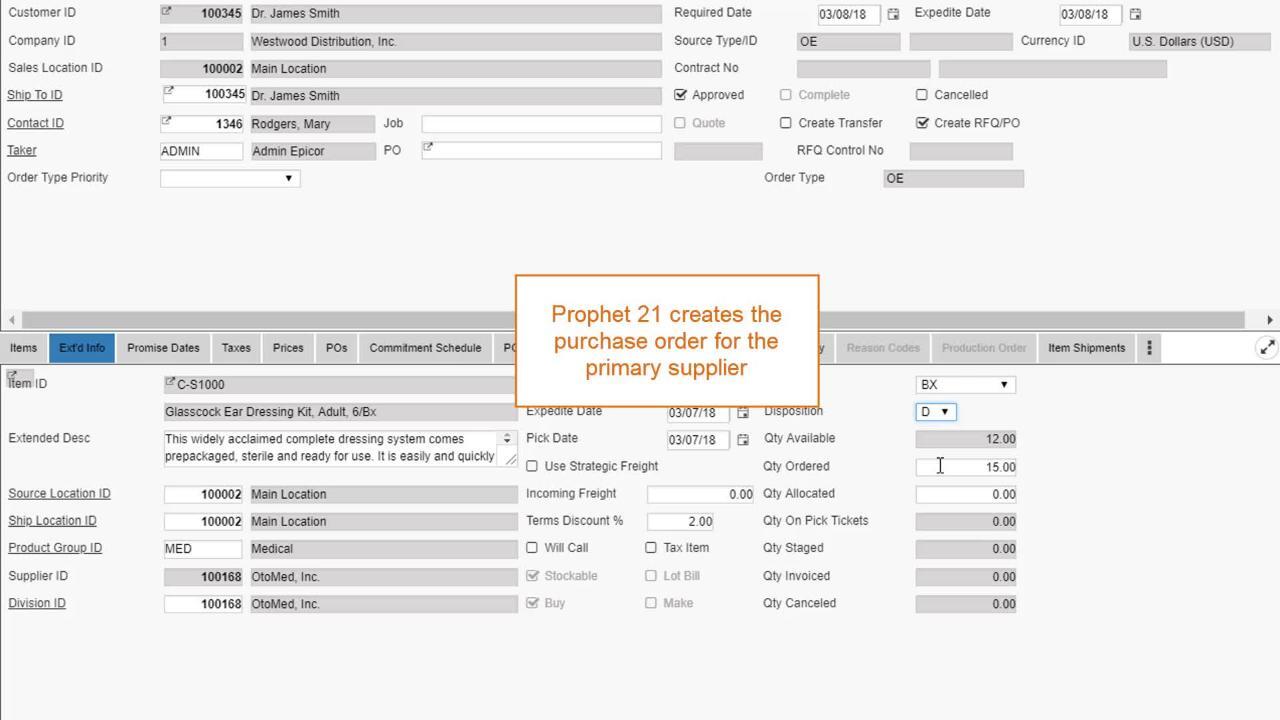Detailed Caption for the Image:

"The image displays a company's purchase order directed to a supplier, showcasing a comprehensive array of details. Prominently featured are the customer IDs, locations, and contact numbers. The document is dated and denotes the source type and supplier ID. Notably, there are checkboxes for 'Approved' and 'Create RFO/PO,' both of which are checked. The order type is specified as OE.

Beneath this section, there is a highlighted segment with a blue and brown box at its center. The text within this box, written in brown, states that 'Profit 21 creates the purchase order for the primary supplier.' The surrounding frame of this section is also outlined in brown.

Further sections of the purchase order continue, detailing it is a medical order. Information about the supplier's name, location, respective discounts, and timelines for order placement and pickup is included. This purchase order exemplifies how 'Profit 21' simplifies the order creation process, enhancing efficiency."